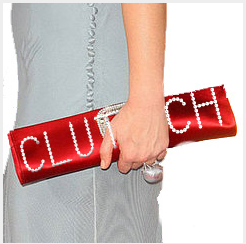The photograph features a woman's torso dressed in a simple gray dress, with visible lines and markings that provide dimensionality with varying shades of gray. The white background starkly highlights her light-skinned forearm and hand, which are holding a slim, rectangular red handbag made of satin. The bag is long and thin, marked by the word "CLUTCH" written in uppercase letters crafted from what appear to be gemstones or pearls. Her thumb is visible as her fingers wrap around the bag, and she wears a large, pearl-like ring on her middle finger. The focus on her minimalist, polished look and the striking red clutch stands out prominently against the monochromatic gray dress and white background.